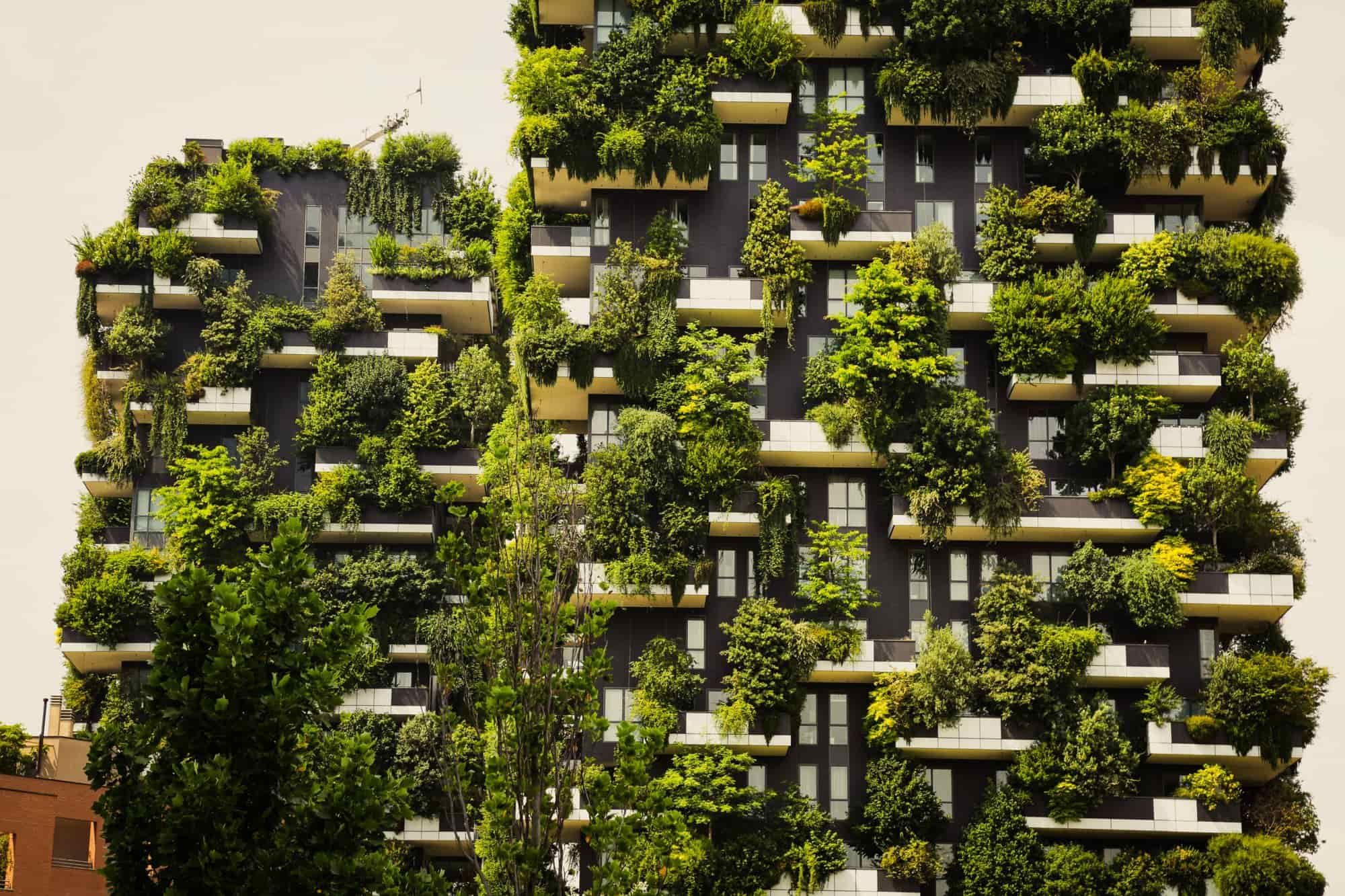This photograph showcases a pair of multi-story buildings that exhibit a unique and striking architectural design. The buildings, predominantly gray, are differentiated by their black facades and staggered white balconies that form a distinct and artistic pattern. The balconies and windows are adorned with various greenery and shrubbery, including overhanging foliage, creating a vivid contrast against the otherwise muted color palette of the scene. Despite the realistic style of the photograph, the abundant and varied green plants give the impression that nature has reclaimed the area, suggesting that the buildings may be abandoned. The daytime setting further highlights the greenery, enhancing the visual impact and emphasizing the diversity of the plant life enveloping this apartment complex. The overall composition, while closely cropped, draws attention to the intricate details of the desolate yet verdant structures.